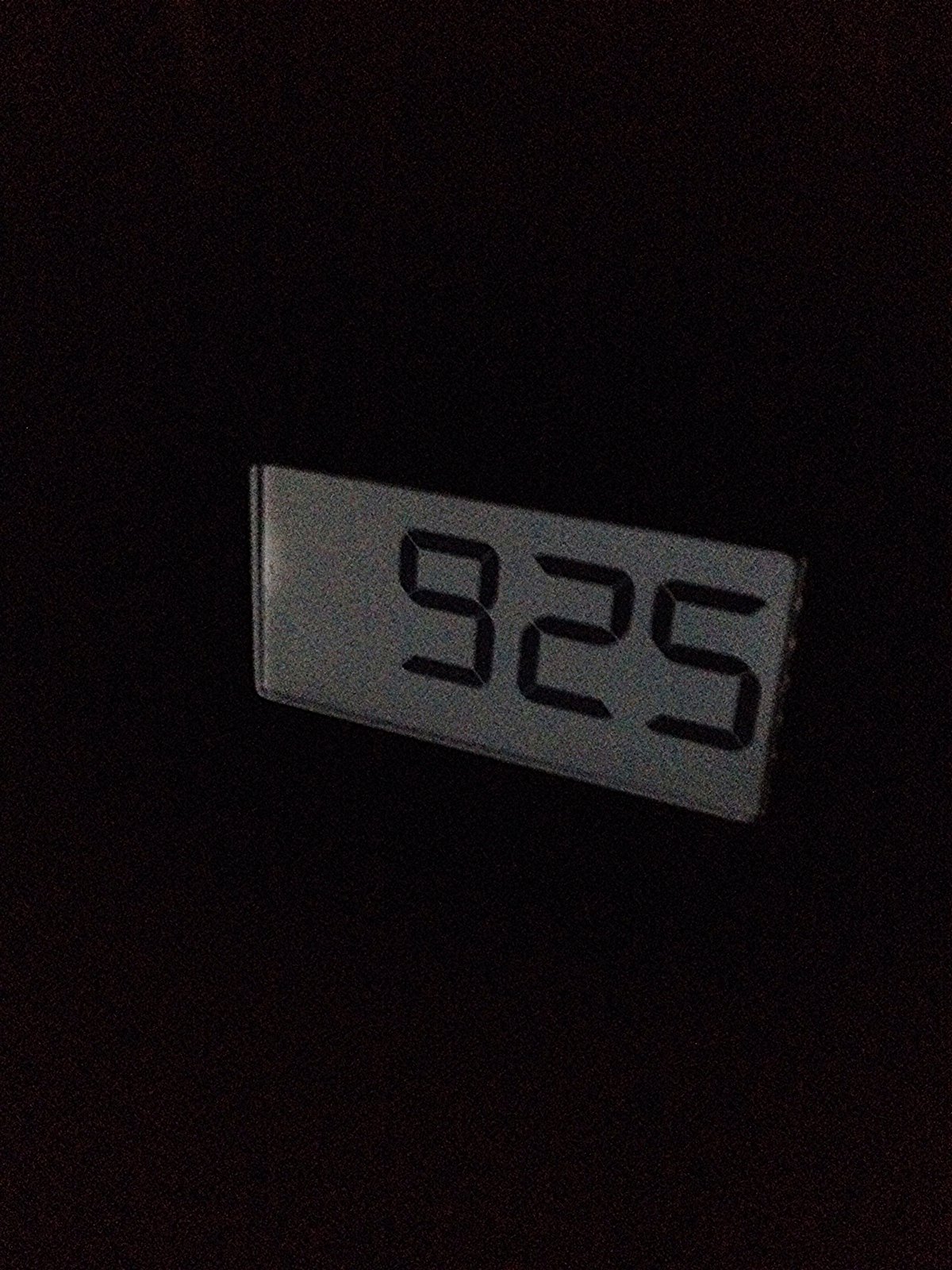The image displays the front face of a digital clock with illuminated numbers set against a textured gray rectangular background. The numbers, reading "925," are positioned towards the top-right corner of the gray rectangle, with the "5" nearly touching the right edge. This gray rectangle, appearing slightly curved at each corner, has a staticky effect composed of numerous tiny colored dots—pink, blue, green, yellow, and orange—giving it a nuanced appearance. The entire image has a vertically rectangular frame, but apart from the gray box, the rest of the background is entirely black without any other visible details or lighting.